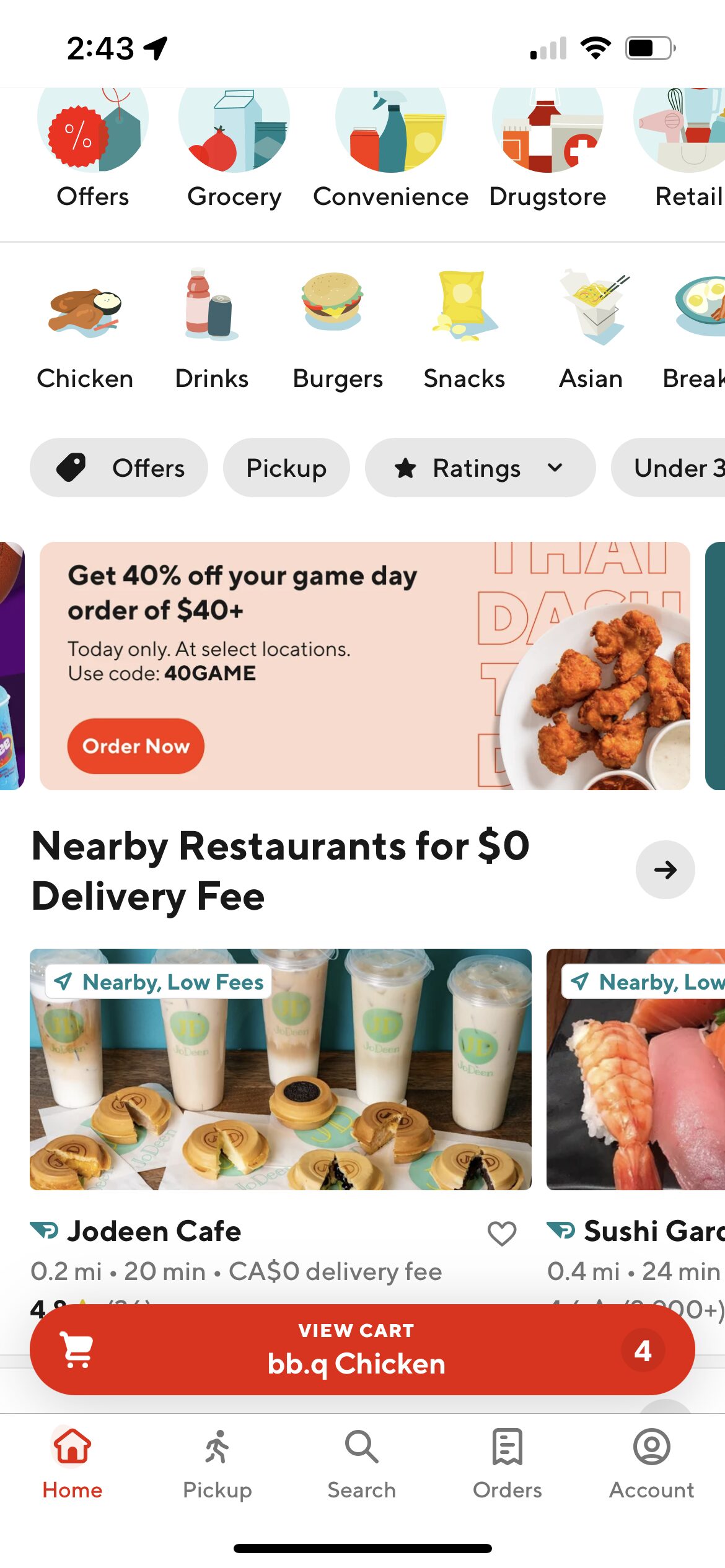Screenshot of a Food Delivery App Interface

This screenshot showcases a food delivery app interface designed for both food and grocery orders. At the top, there are various icons representing different options such as "Offers," "Grocery," "Convenience," "Direct Store," and "Retail." The time on the phone is 2:43, and the status bar indicates a single bar of network signal, a Wi-Fi connection, and about half battery life remaining.

Below the top options, there are additional icons representing different types of food choices, including "Chicken," "Drinks," "Burgers," "Snacks," and "Asian." The "Breakfast" icon is partially cut off. Underneath these, there are clickable icons in gray with black font that read "Offers," "Pickup," and "Ratings Under 3."

A prominent ad appears below these options, featuring a pink background and an orange "Order" button. The ad promotes a deal offering "40% off your game day order of $40+" with a coupon code "40GAME." The ad includes a tempting image of chicken wings on a plate with dipping sauces.

Further down, the app highlights nearby restaurants offering a $0 delivery fee, with an arrow prompting users to explore more options. Directly beneath this is an ad for Jodine Cafe, located 0.2 miles away, displaying its delivery fee and a clickable "View Cart" button in orange. The cart contains four items, including BBQ chicken.

At the bottom of the screen, the menu bar contains five options: "Home," "Pickup," "Search," "Orders," and "Account." The "Home" button is highlighted in orange, while the other options are in gray.